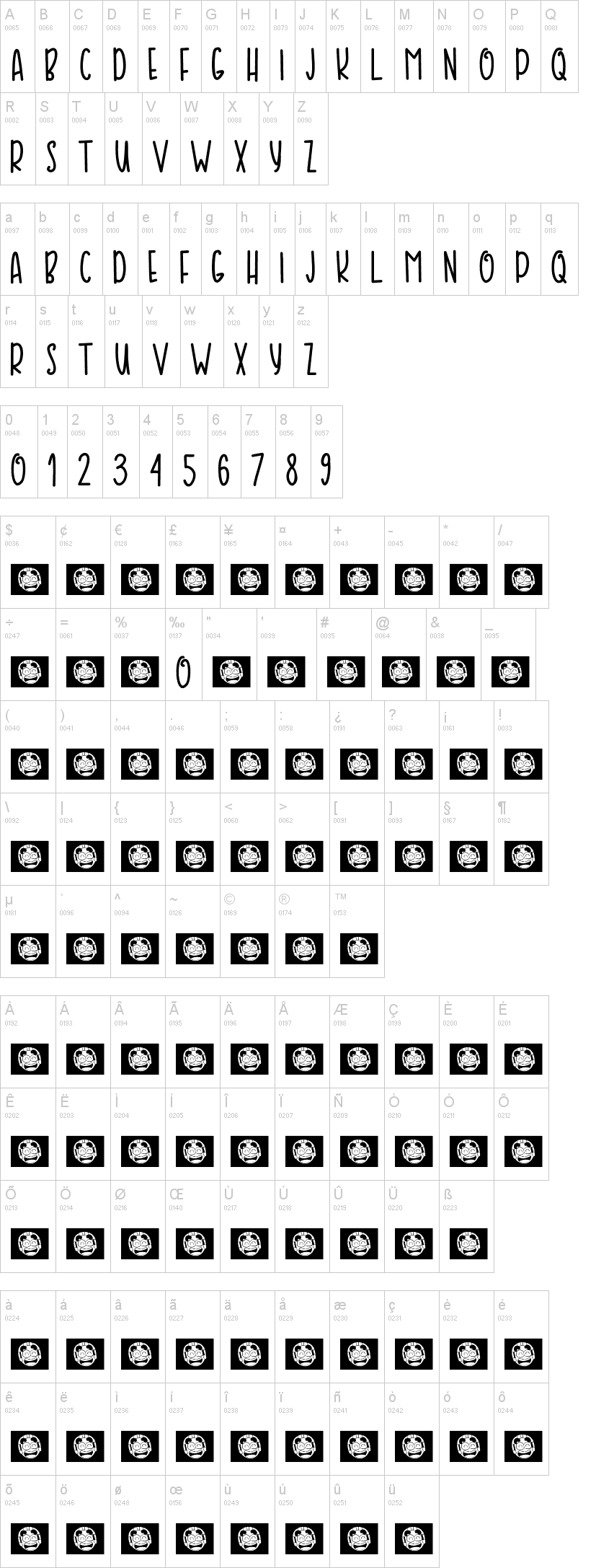The image features a white background with distinct sections. At the top part, uppercase letters A through Z are written in black, alongside their respective ASCII codes, ranging from 0065 (for A) to 0090 (for Z). Directly below, there is a second row that displays lowercase letters a through z with their corresponding ASCII codes, starting from 0097 (for a) and ending at 0122 (for z).

Additionally, a row featuring numbers 0 through 9 is present, with each number accompanied by its ASCII code, starting at 0048 (for 0) and ending at 0057 (for 9). Following this, special characters begin with the dollar sign ($) and its ASCII code 0036, progressing through a series of characters, concluding with the trademark symbol (™) and its ASCII code 0153.

Moreover, a separate section showcases accented uppercase characters, starting from 0192 and ending at 0223. Lastly, there is a collection of accented lowercase characters whose ASCII codes range from 0224 to 0252.